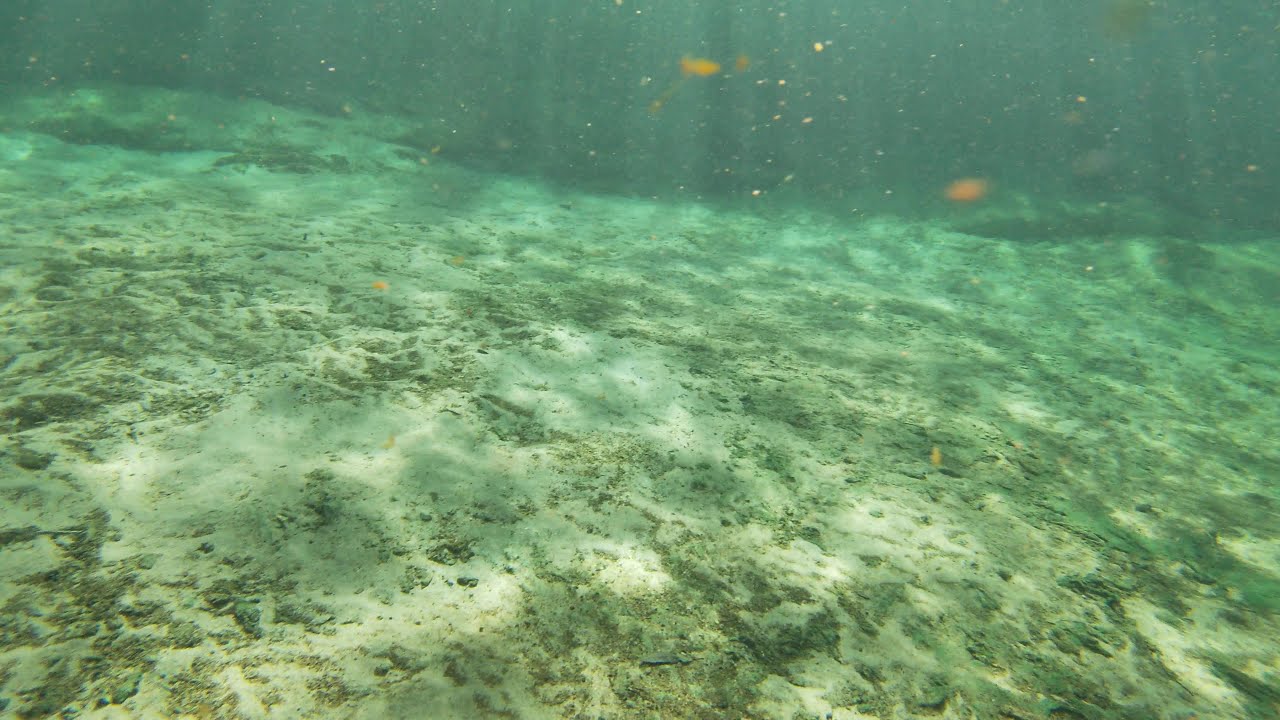This underwater image captures the tranquil yet dynamic nature of a shallow ocean floor. The photograph predominantly showcases a sandy surface sprinkled with rocky debris and sediment, reflecting a mix of tan, brown, green, blue, orange, and yellow hues. The water above appears slightly murky, with visible floating particles and sediment, adding to the natural authenticity of the scene. Sunlight streams through the water, creating vertical beams and delicate wavy patterns on the ocean floor, enhancing the overall ambience with bright patches interspersed with darker teal shadows. Far in the background, there are faintly discernible orange fish, adding life to this serene snapshot of the underwater world.